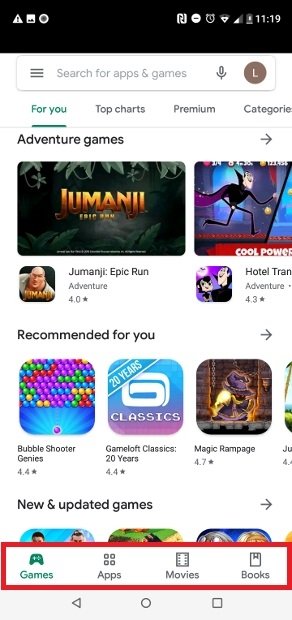The smartphone screenshot taken at 11:19 AM displays the status bar with an alarm clock icon, a Wi-Fi icon showing two signal bars, and battery status. Below the status bar, there's a search box with the placeholder text "Search for apps and games," featuring a hamburger menu icon on the left, a microphone icon on the right, and a brown circle with the letter "L" next to the microphone icon. 

Further down, the main interface categorizes sections labeled as "For You," "Top Charts," "Premium," and "Categories." Under these tabs, the screenshot highlights a section titled "Adventure Games" featuring a thumbnail for "Jumanji: Epic Run" which is classified as an adventure game with a 4.0 rating.

Adjacent to the Jumanji game thumbnail, there's another game thumbnail that depicts a vampire character. Below these, the section "Recommended for You" is displayed with games such as "Bubble Shooter," "Gameloft Classics: 20 Years," and "Magic Rampage." The bottom part of the screenshot showcases the section labeled "New and Updated Games."